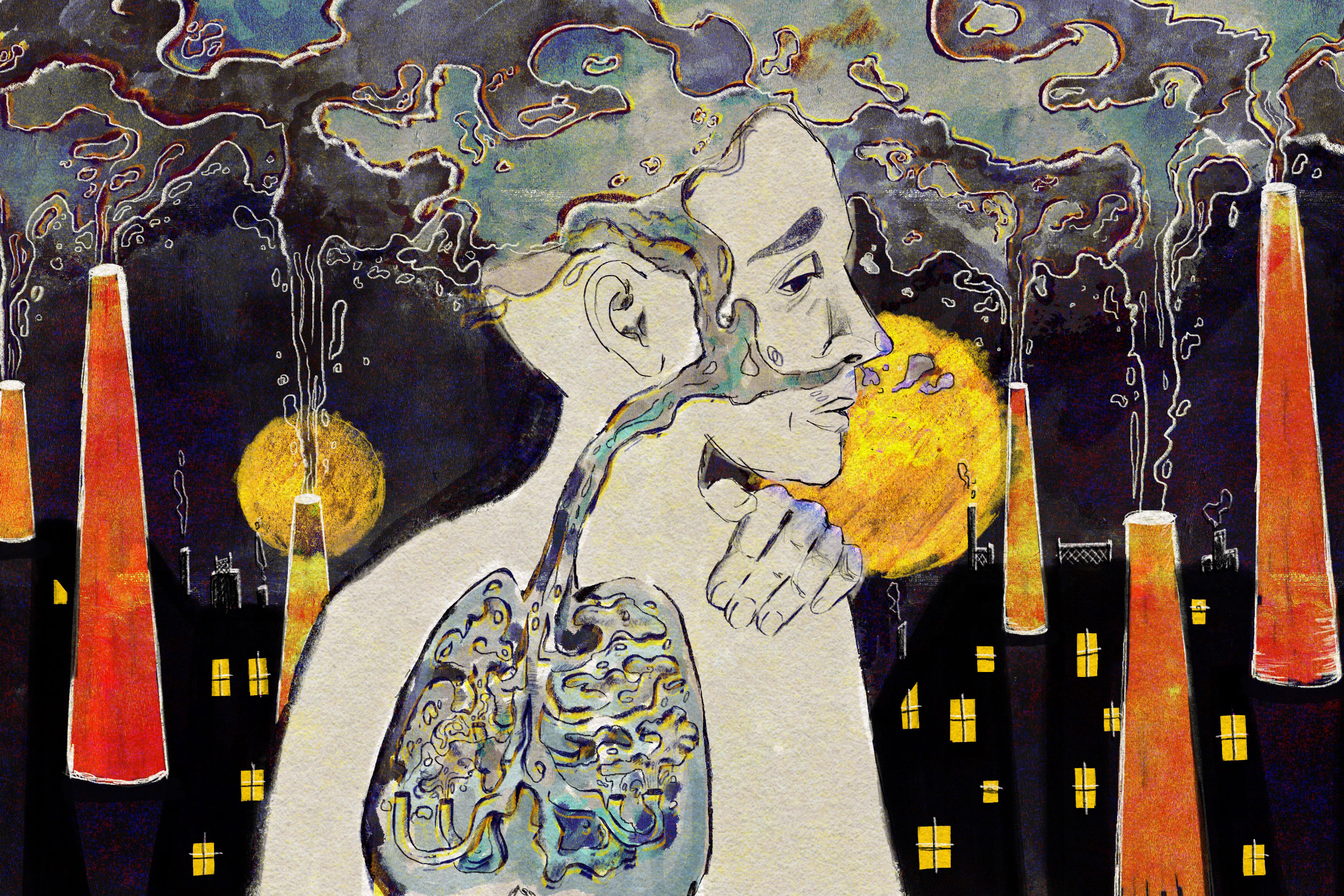This surreal painting depicts a male figure set against a nighttime cityscape with buildings featuring yellow-lit windows. The man's profile, facing right, is outlined in white with intricate detailing on his face and a hand resting on his right shoulder from an unseen person. The figure’s torso reveals a detailed view of his nervous system and lungs, which are portrayed using shades of gray. Swirling clouds of smoke emerge from his lungs and ascend through the top of his head, which appears to be partially opened or removed. These plumes of smoke integrate with those emanating from various bottles and orange chimneys scattered throughout the scene, all converging in a complex, swirling pattern. The background features a deep black sky with two distinct orange moons, one larger than the other, enhancing the surreal and haunting atmosphere of the image. The painting uses a blend of bold colors like orange, blue, and yellow to highlight elements like the bottles and smoke, creating a vivid contrast against the otherwise monochromatic elements of the figure and cityscape.